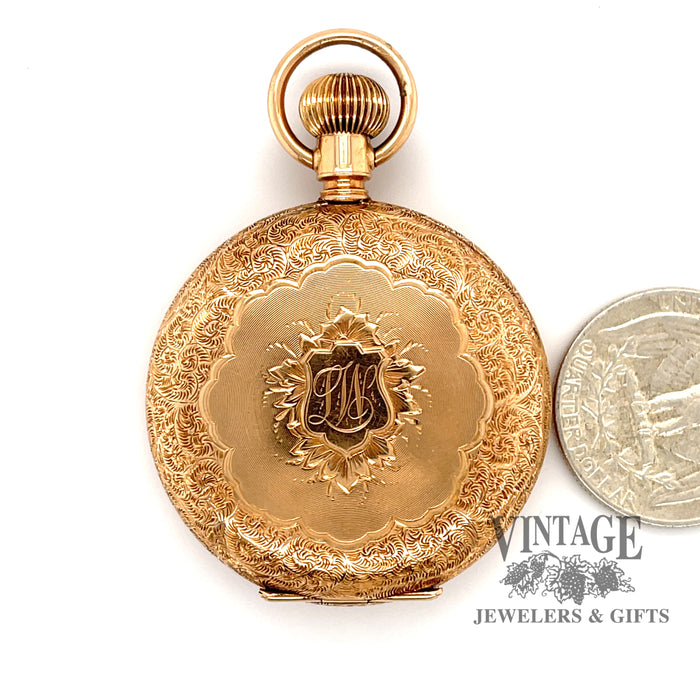The image features a detailed, old-fashioned pocket watch prominently centered against a solid white background. The watch, made from shiny gold metal, is intricately designed with ornate fern leaf and floral patterns etched around its round shape. At the center of its smooth metal surface, there's a shield-like emblem adorned with the cursive initials "LW" encircled by petal-like designs and stemming leaves. A small clasp latch at the bottom indicates where the watch can be opened, and a circular ring at the top with a central ball and vertical lines suggests the point for adjusting the time. Positioned to the right of the pocket watch is a quarter, included to provide a sense of scale. The lower right corner of the image features a black and gray watermark logo that reads "Vintage Jewelers and Gifts," hinting that this may be an advertisement for the business, likely intended for their website.